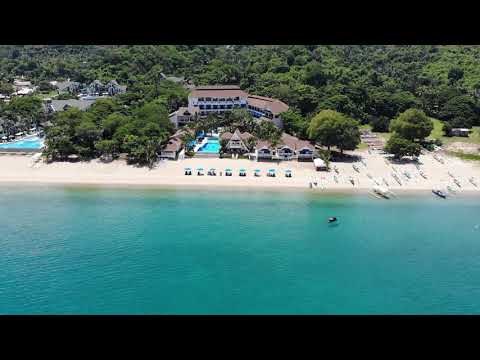This drone shot captures an expansive aerial view of a vibrant beach resort. At the heart of the image stands a large hotel with multiple brown-roofed buildings, surrounded by lush green trees that dominate the background. The hotel features several pools scattered around its premises, with additional resort buildings visible on the left. In the very center, a row of blue umbrellas shelters numerous beachgoers relaxing beneath them. To the right, people are either bringing in or taking out boogie boards and kayaks to the sandy shore, which transitions into crystal clear, azure ocean waters. Despite the image being somewhat pixelated and grainy, one can still discern the lively atmosphere of this inviting vacation spot.